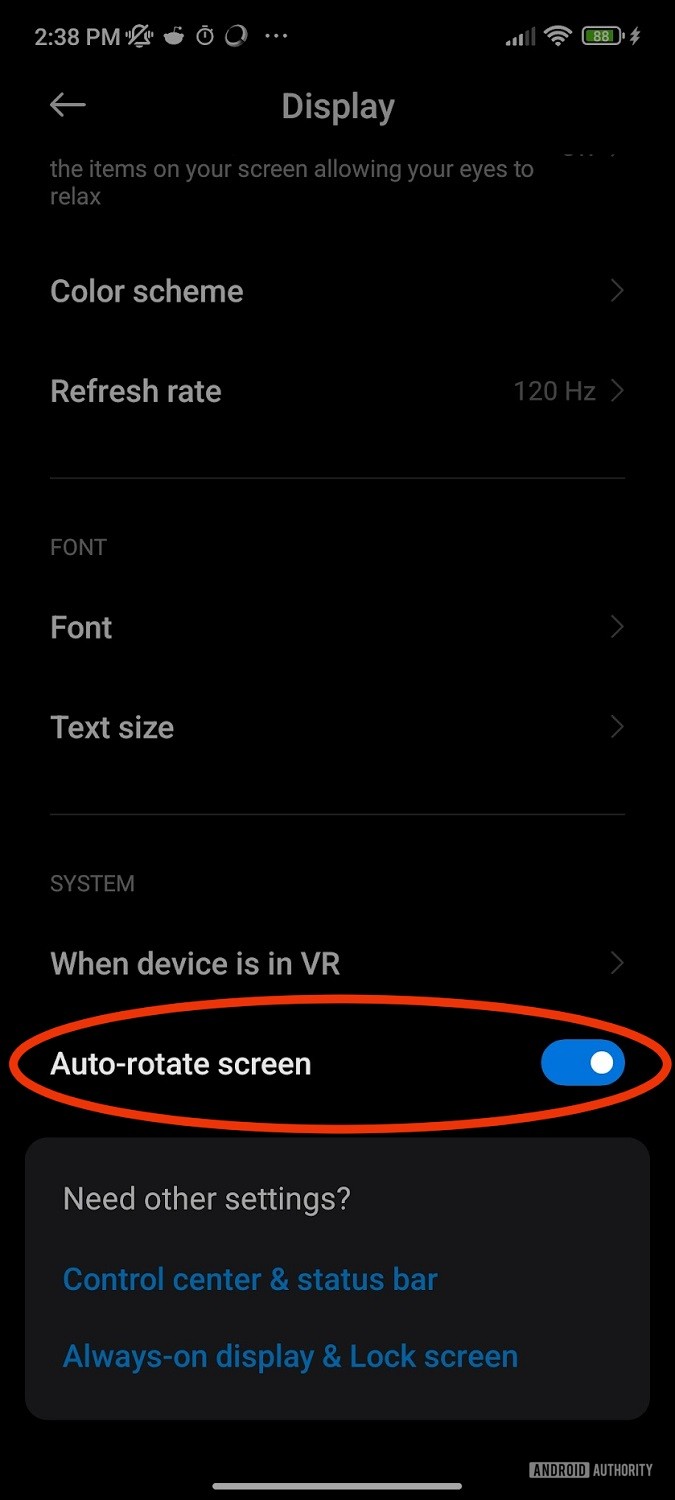The screenshot depicts a settings screen from a mobile device, potentially a tablet or a phone. The background is black with all the options listed in white text for easy readability.

At the top center of the screen, the heading reads "Display." Directly below it is a descriptive line that says, "The items on your screen, allowing your eyes to relax." Below this are various adjustable settings:

1. **Color Scheme**: This option has a clickable arrow to the right, which likely leads to additional settings.
2. **Refresh Rate**: Listed at "120 Hz," this setting also has a clickable arrow beside it for further customization options.
3. **Font** (fainter text): This section includes two options:
   - **Font Style**
   - **Text Size** Each of these has a clickable arrow to the right for additional settings.

Further down, under the fainter heading **System**, there are more options:
4. **When device is in VR**
5. **Auto Rotate Screen**: This option is active, as indicated by a blue slider button to the right. Notably, this entire option is circled in orange for emphasis.

At the very bottom, in a fainter gray text, is a section asking, "Need other settings?" followed by:
- **Control Center and Status Bar** (highlighted in blue)
- **Always On Display and Lock Screen** (also highlighted in blue)

Every element on this settings screen is intuitively designed to enhance user interaction and eye comfort.